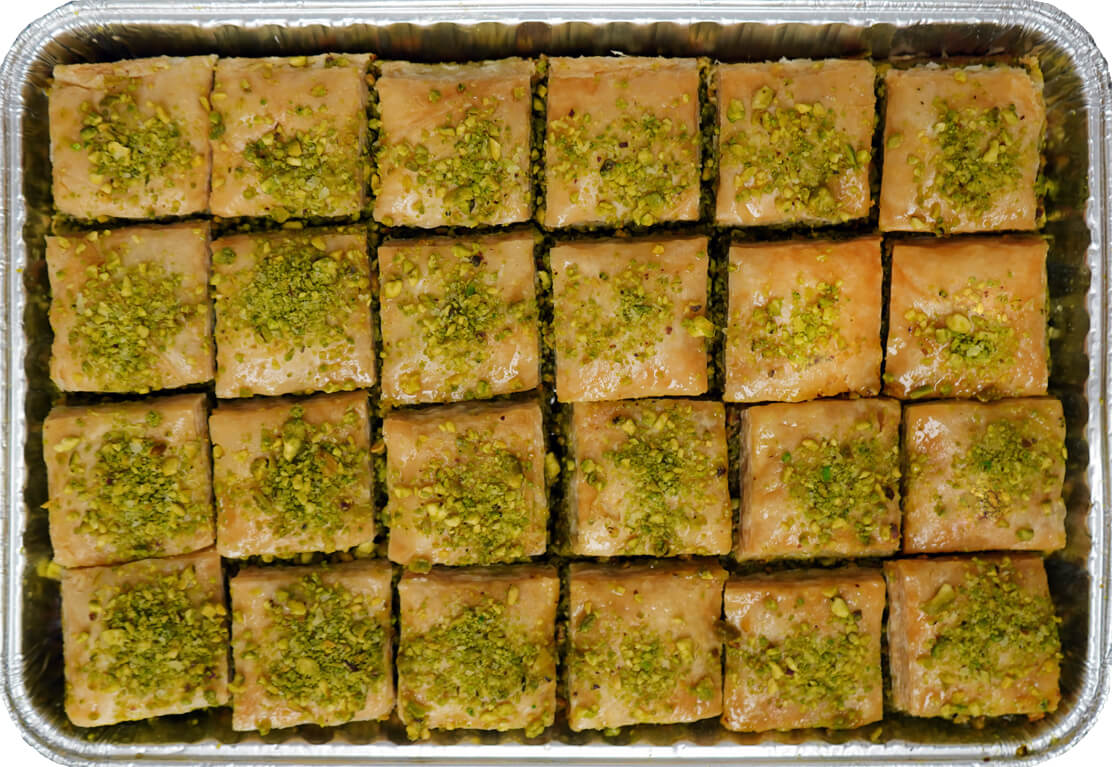This top-view, color photograph in landscape orientation showcases a rectangular, disposable aluminum foil baking tin with curved corners. The silver-colored tin, floating against a white background, contains 24 neatly arranged squares of baklava, laid out in organized rows and columns—4 rows by 6 columns. The baklava squares feature golden pastry tops and are generously sprinkled with finely chopped green pistachio nuts. The texture reveals a tan, granular, crust-like surface indicative of the baked pastry dessert, exuding a slightly moist appearance where the pistachios are. The photograph combines elements of realism and representationalism, capturing the intricate details of the dessert in a style true to food photography.